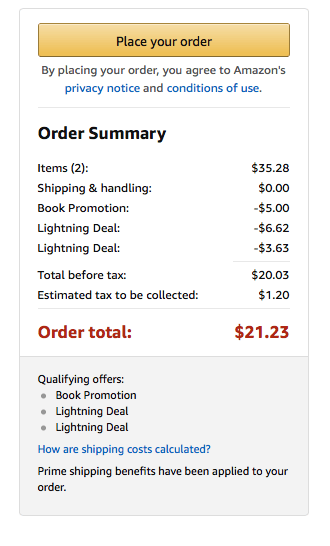Screenshot of Amazon's 'Place Order' section featuring a prominent yellow 'Place Your Order' button at the top. Below it, a message reads, "By placing your order, you agree to Amazon's Privacy Notice and Conditions of Use." The order summary details are as follows: 

- Items (2): $35.28
- Shipping and Handling: $0.00
- Book Promotion: -$5.00
- Lightning Deal 1: -$6.62
- Lightning Deal 2: -$3.63

Total before tax: $20.03
Estimated tax to be collected: $1.20
Order total: $21.23

The screenshot also highlights qualifying offers, including book promotions and lightning deals, along with a note explaining how shipping costs are calculated. At the bottom, it confirms that "Prime shipping benefits have been applied to your order."